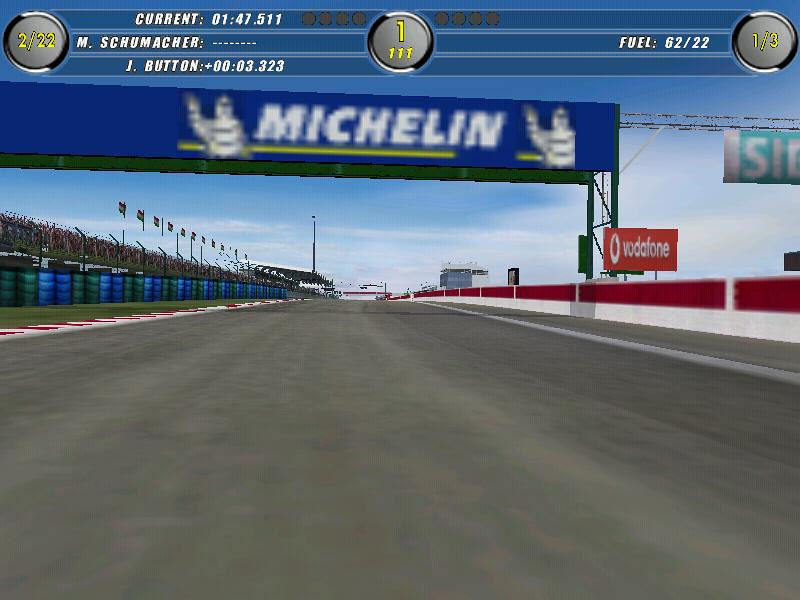The image depicts a scene from a racing computer game. At the top of the screen are three buttons, each displaying important in-game information. The button on the left shows "2/22" in yellow font, indicating the current lap out of a total of 22 laps. The center button displays the number "1" alongside three symbols, possibly representing the player's position or status indicators such as speed, gear, or special abilities. The button on the right reads "1/3" in yellow font, possibly denoting the position out of a total of three players or cars.

The main focus of the image is a detailed raceway or track. On the right side of the track is a white wall adorned with black and red sections, which may be marking or branding elements on the track. From the right edge of the screen, a black object can be seen entering the frame, potentially another vehicle or track-related equipment, contributing to the dynamic nature of the racing scene.